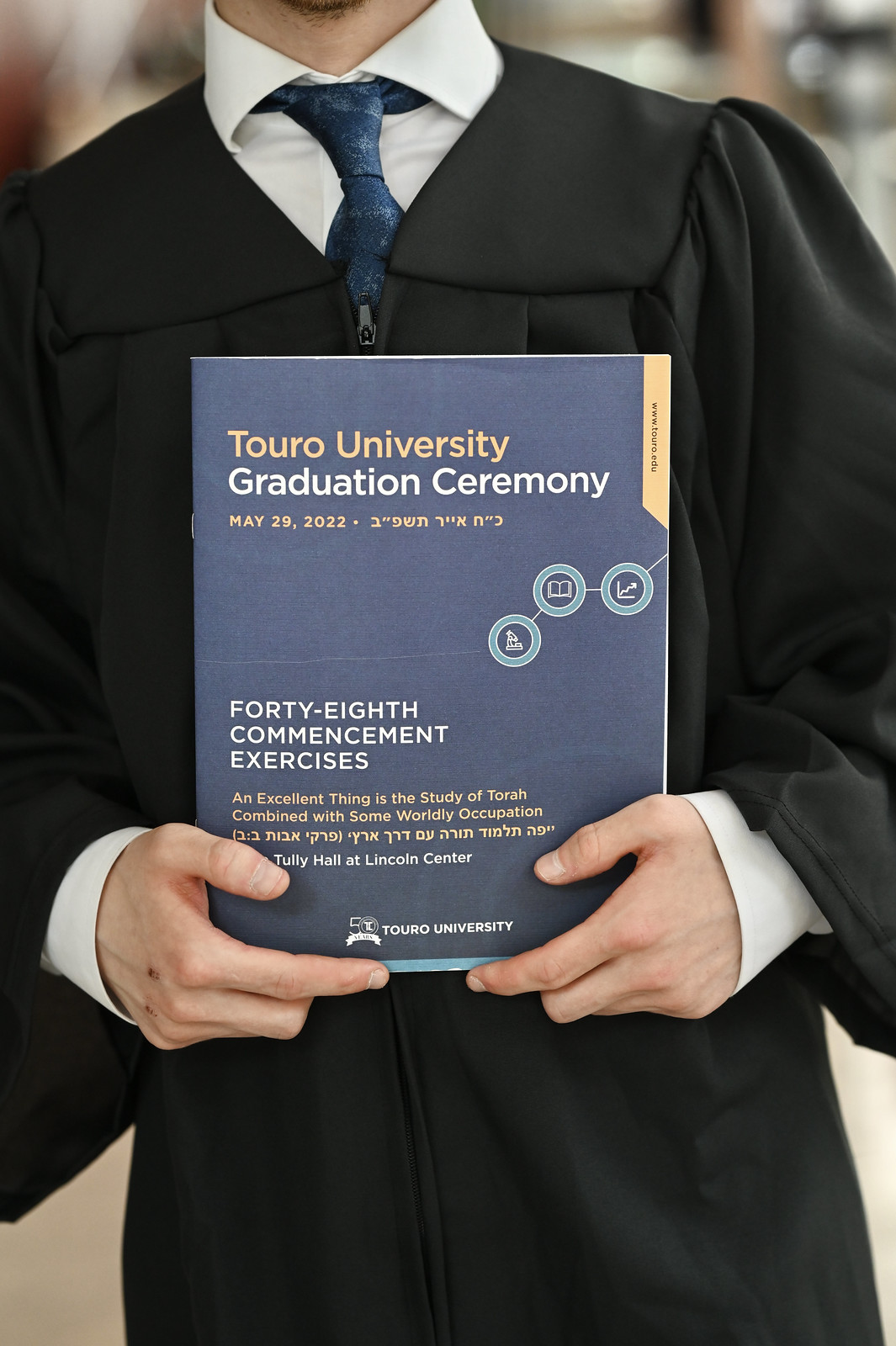In this detailed photograph, the frame captures the torso of a person dressed in full graduation attire, extending from their neck down to just below their waist. The individual is dressed in a traditional graduation gown, beneath which they are wearing a crisp white shirt and a neatly knotted blue tie. The person's hands are prominently visible, firmly gripping a blue program booklet. 

The cover of the booklet prominently features the words "Touro University Graduation Ceremony" at the top, followed by the date "May 29th, 2022." Further down, the booklet highlights the "48th Commencement Exercises" and includes the quote, "An excellent thing is the study of Torah combined with some worldly occupation." The bottom portion of the cover includes the location, "Tully Hall at Lincoln Center," and the name "Touro University," repeated for emphasis. Additionally, there is a small amount of text in an unidentified Asiatic script, adding an international flair to the occasion. The surrounding details and the clear text on the booklet emphasize the importance and ceremonial nature of this significant academic achievement.